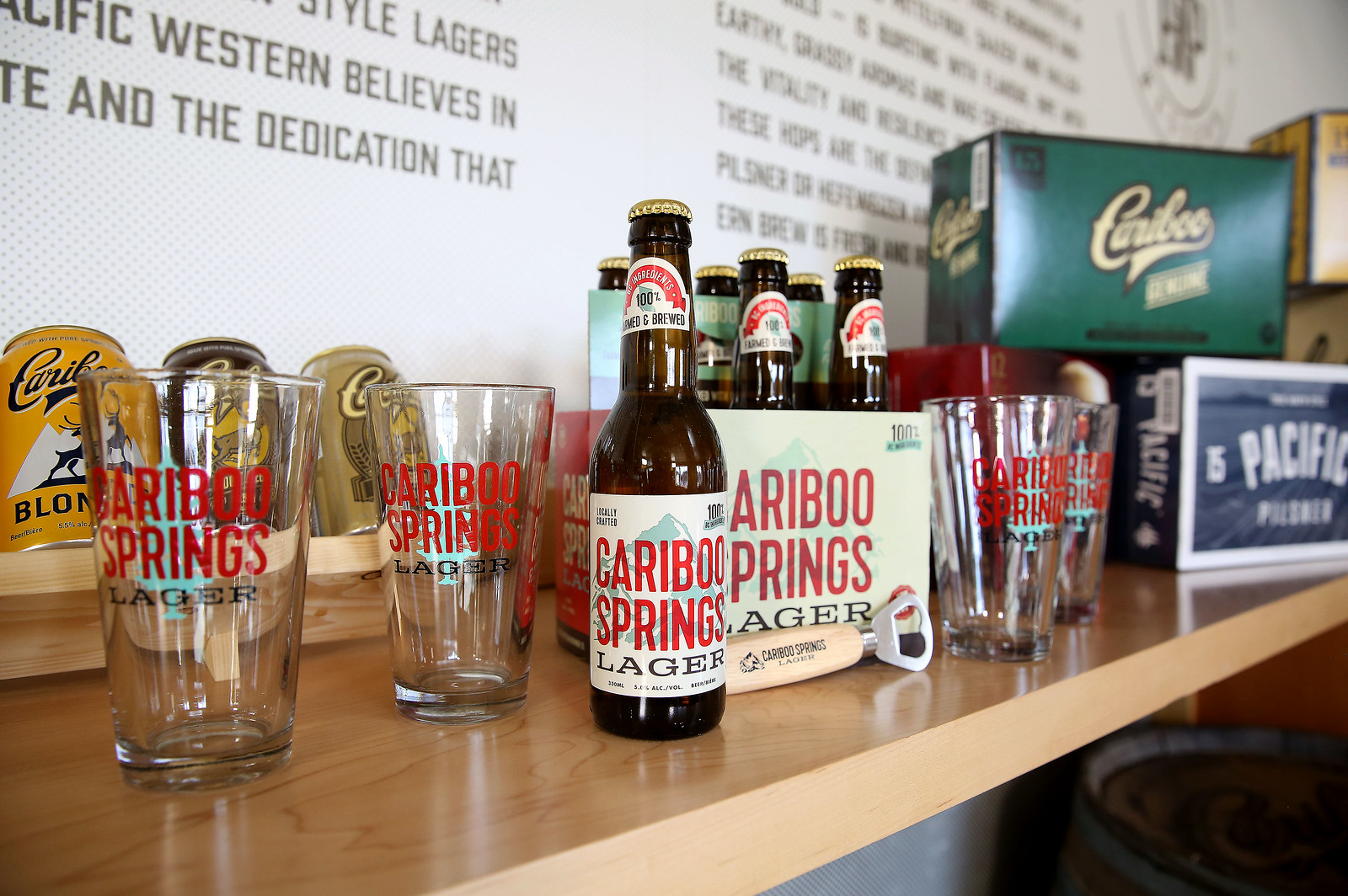The photograph captures a bar scene featuring Caribou Springs Lager. Four empty pint glasses, each branded with "Caribou Springs" in red font and "LAGER" in black capital letters, are symmetrically arranged—two on the left and two on the right. Centered slightly to the right is a six-pack of Caribou Springs Lager, with one bottle displayed prominently in front. This bottle's label highlights "Locally crafted" and "5.0% alcohol per volume" with a mountain graphic in the background. To the left of the six-pack, a wooden-handled bottle opener features the Caribou Springs Lager branding. Further in the background, the bar is lined with various colored beer cases—green, blue labeled "Pacific," yellow, and red—all bearing the Caribou logo. Additionally, a wooden display on the left side showcases three different Caribou beer cans in yellow, black, and tan. The overall setting suggests a bar or brewery, with additional wall text that is partially readable.